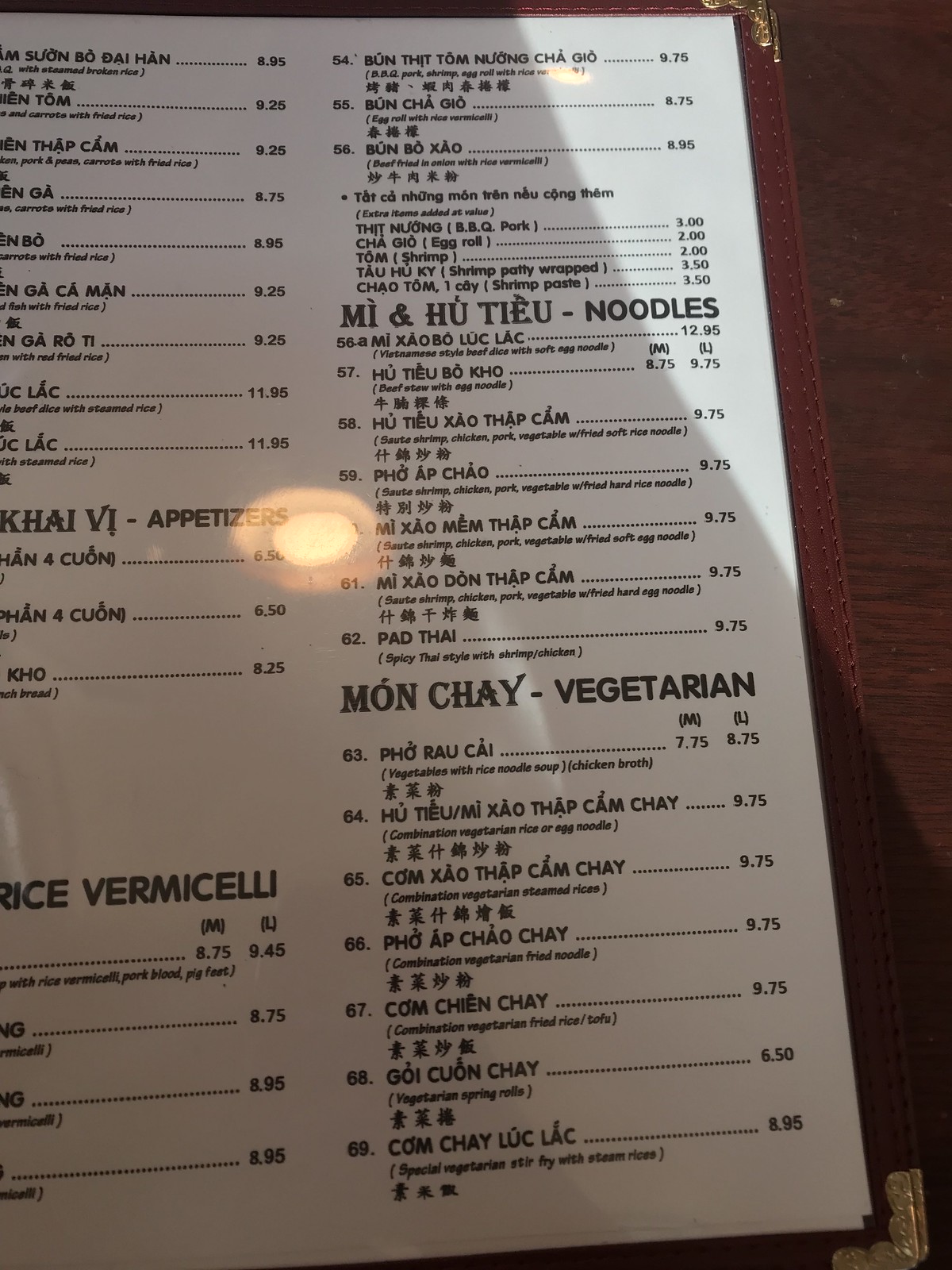The image features a bilingual menu in both Vietnamese and English. Dominating the right side of the image are pictures of various noodle dishes. The Vietnamese text and characters are prominently displayed at the top of each section, followed by the English translations underneath. 

The menu includes:

- **Vietnamese-Style Beef**: Sliced beef served with soft egg noodles for $12.95.
- **Beef Stew with Egg Noodle**: A hearty option listed among the selections.
- **Various Satay Dishes**: Options include shrimp, chicken, pork, and vegetables, which can be paired with:
  - Fried soft rice noodles
  - Fried hard rice noodles
  - Fried soft egg noodles
  - Fried hard egg noodles

Additionally, there is a **Spicy Thai-Style Pad Thai** featuring tripret chicken.

In the vegetarian section, a range of dishes is offered with prices differentiated by portion size: medium for $7.75 and large for $8.75.

Overall, the menu provides a detailed and diverse selection of both meat-based and vegetarian Vietnamese dishes.